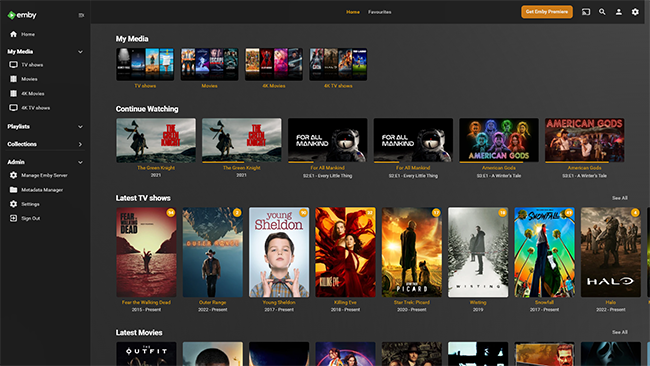The website displays a black background with a white navigation menu on the left-hand side. The top entry bears the initials "MB" in white. As the text is quite small and becomes blurry when zoomed in, it is difficult to decipher all the entries clearly. The menu likely starts with "Home," followed by possibly "My Media." The next entry could be "TV Shows" or something similar, although it is not entirely discernible.

Further down, the menu may contain an entry labeled "4K TVs" or related to 4K content, and another labeled "Playlists." Below that, it reads "Collections" and "Admins." Adjacent to or below these entries is a section marked with an "M," possibly indicating "Manager" or a similar term. Lower on the menu, there is an option for "Settings" and a "Sign Out" button.

On the main area of the site, highlighted entries in yellow for easier visibility include "My Media," "TV Shows," and "Movies," alongside what reads as "4K Movies" and "4K TV Shows." There are listings of content as well, such as "The Green Knight," "For All Mankind," and "American Gods" (appearing twice). Below these, a section labeled "Latest TV Shows" lists titles, including "Fear the Walking Dead" and "Young Sheldon." Some titles and words remain unclear due to the blurriness when zoomed in.